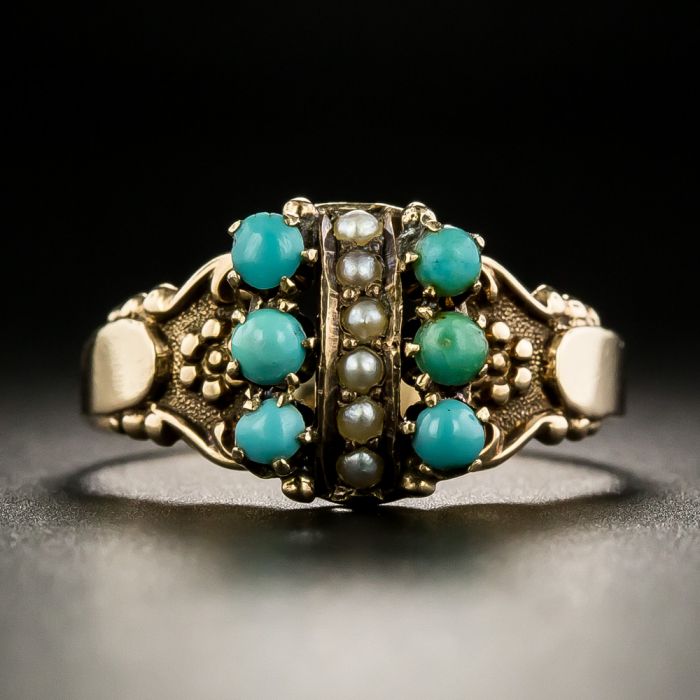The image displays a close-up of a stylish piece of jewelry, likely a ring, with a striking gold hue, though it may not be real gold. The ring is set against a black and grey background which enhances its prominence. The ring features an intricate design with numerous details; it has small floral motifs intricately carved into the metal. The centerpiece includes six luminescent, off-white pearls arranged vertically, flanked by three teal-colored stones on each side. The stones appear to be turquoise beads, offering a contrast with the gold's warmth. The light source from behind creates a subtle glow and a circular reflection beneath the ring, emphasizing its detailed craftsmanship and elegant form.